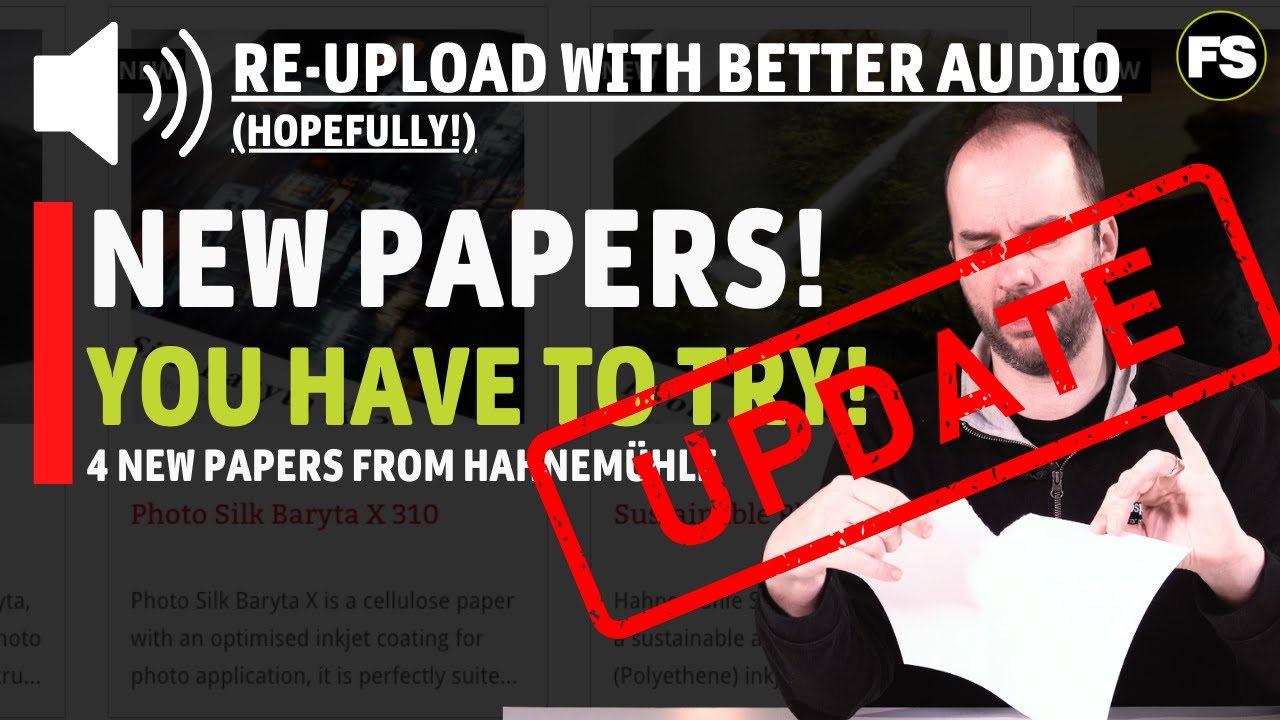The image appears to be a video thumbnail, possibly for a YouTube video, about re-uploading with improved audio quality. Dominating the top left corner is a white megaphone icon with sound waves, alongside text that reads "Re-upload with better audio (hopefully)!" Below this, in bold letters, it says "New papers! You have to try!" In smaller text, it mentions "Four new papers from H-A N-E-M-U-H-L with an umlaut," though part of this text is obscured. A large red stamp with "UPDATE" covers part of the screen, superimposed on an image of a man on the right side. The man, who has balding dark hair, a beard, stubble, and a mustache, is dressed in black while ripping a piece of white paper. Additionally, the upper right-hand corner features a yellow circle with the letters "F.S." and the background shows text related to "Photosilk Barada X310" and optimized inkjet coating for cellulose paper.